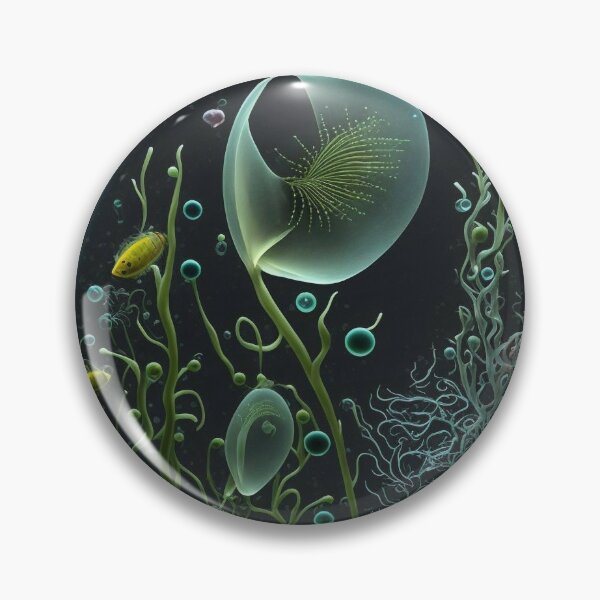The image showcases a detailed 3D digital art design with a central black circular object. This circle, resembling a button or a glass piece, contains an intricate scene of aquatic life and exotic, alien-like plants. Inside the circle, there's a yellow fish positioned towards the left, middle section, surrounded by other sea creatures and vibrant plant life. The plants exhibit a variety of colors including green, blue, turquoise, yellow, and teal. Bubbles, appearing bright teal, enhance the underwater effect, while a large, light teal flower with yellow lines stands out as the most prominent shape. The background inside the circle is strikingly black, contrasting sharply with the empty white space that surrounds the circle, making the central design appear even more vivid. The overall image is framed within a square, with no text present to distract from the visual artistry.